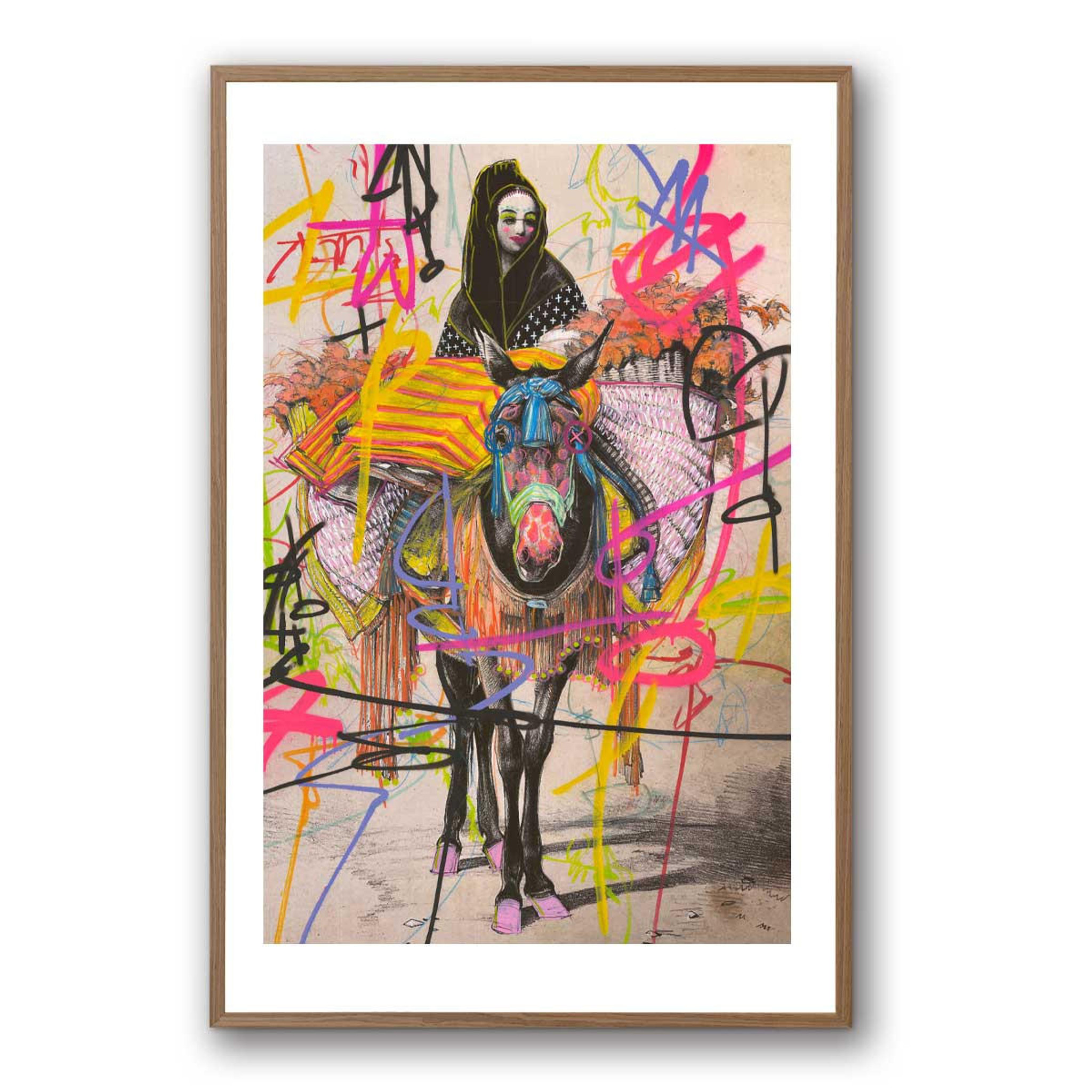This photograph captures a framed artwork that juxtaposes vintage and contemporary styles. The frame is slender, wooden, and unadorned, while the white matting sets a clean border around the rectangular piece, which is taller than it is wide. At the center is a black-and-white photograph of a woman, possibly of Asian or Mexican descent, wearing a black robe and headscarf. She sits atop a horse laden with large woven baskets brimming with flowers. The original image is formal and posed, yet has been exuberantly transformed with vibrant graffiti-style art. The horse features pink hooves, a blue scarf across its forehead, a green bit, and pink dots forming a zebra-like pattern on its face. The woman has been given cartoonish rosy cheeks and sunglasses in the modern overlay. The entire scene is overlaid with a riot of spray-painted colors—pink, yellow, black, and blue—forming random squiggly lines, symbols, and even a heart, creating an eye-catching fusion of the old and new.